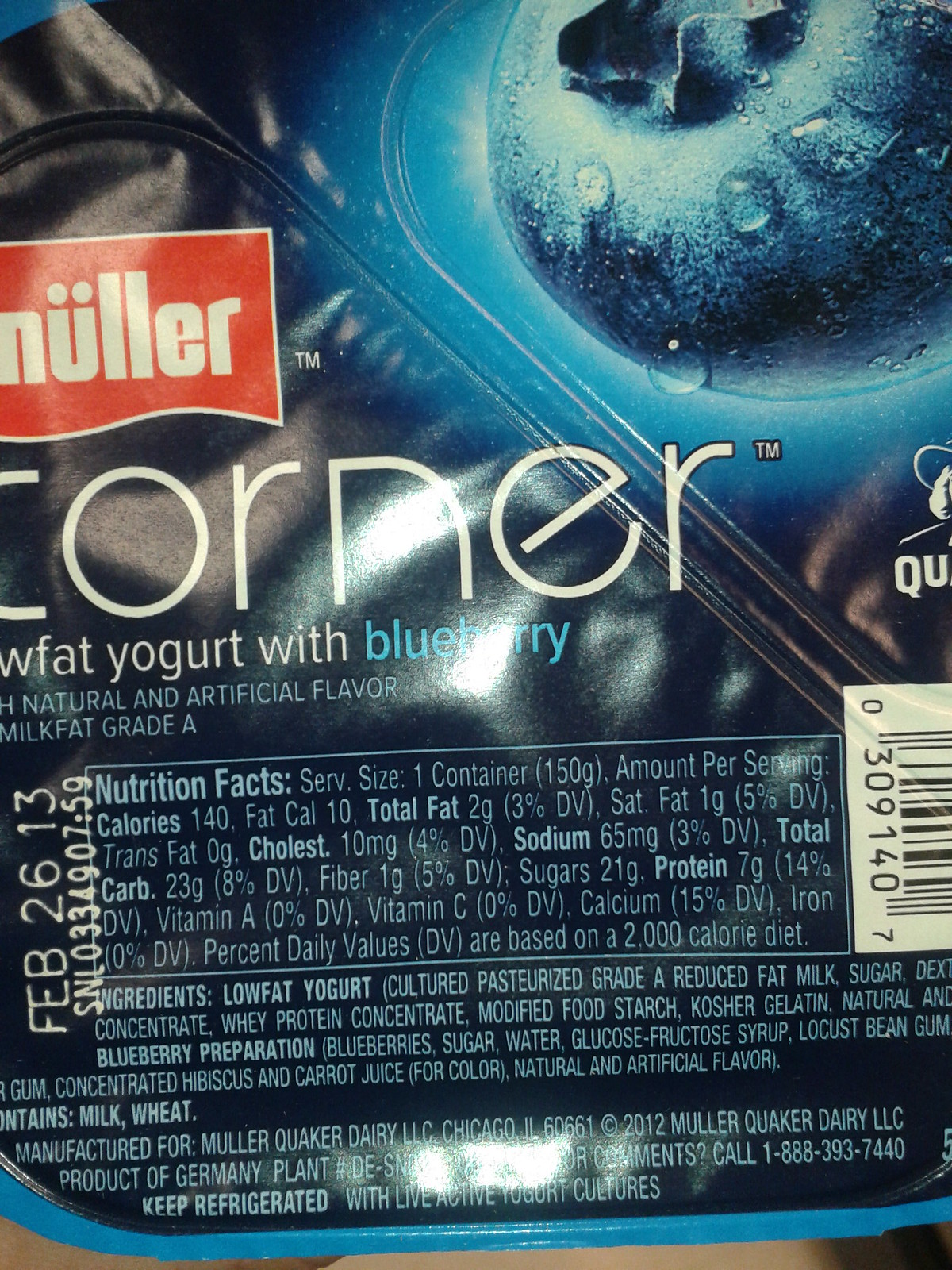This extreme close-up image features a food product label with a distinct dark blue and light blue color scheme. Dominating the label is a prominent image of a blueberry, set against the lighter blue backdrop. The manufacturer's logo, "Knoller," stands out, guiding the eye to the product description that reads: "Corner, Low-Fat Yogurt with Blueberry," complemented by additional details such as "with natural and artificial flavor" and "milk fat grade A," all in crisp white text. The label also includes a barcode and a nutrition facts table, neatly positioned at the bottom. The expiration date clearly states "February 26, 2013." Below the nutrition facts, the label lists the ingredients and provides a contact phone number for the manufacturer.